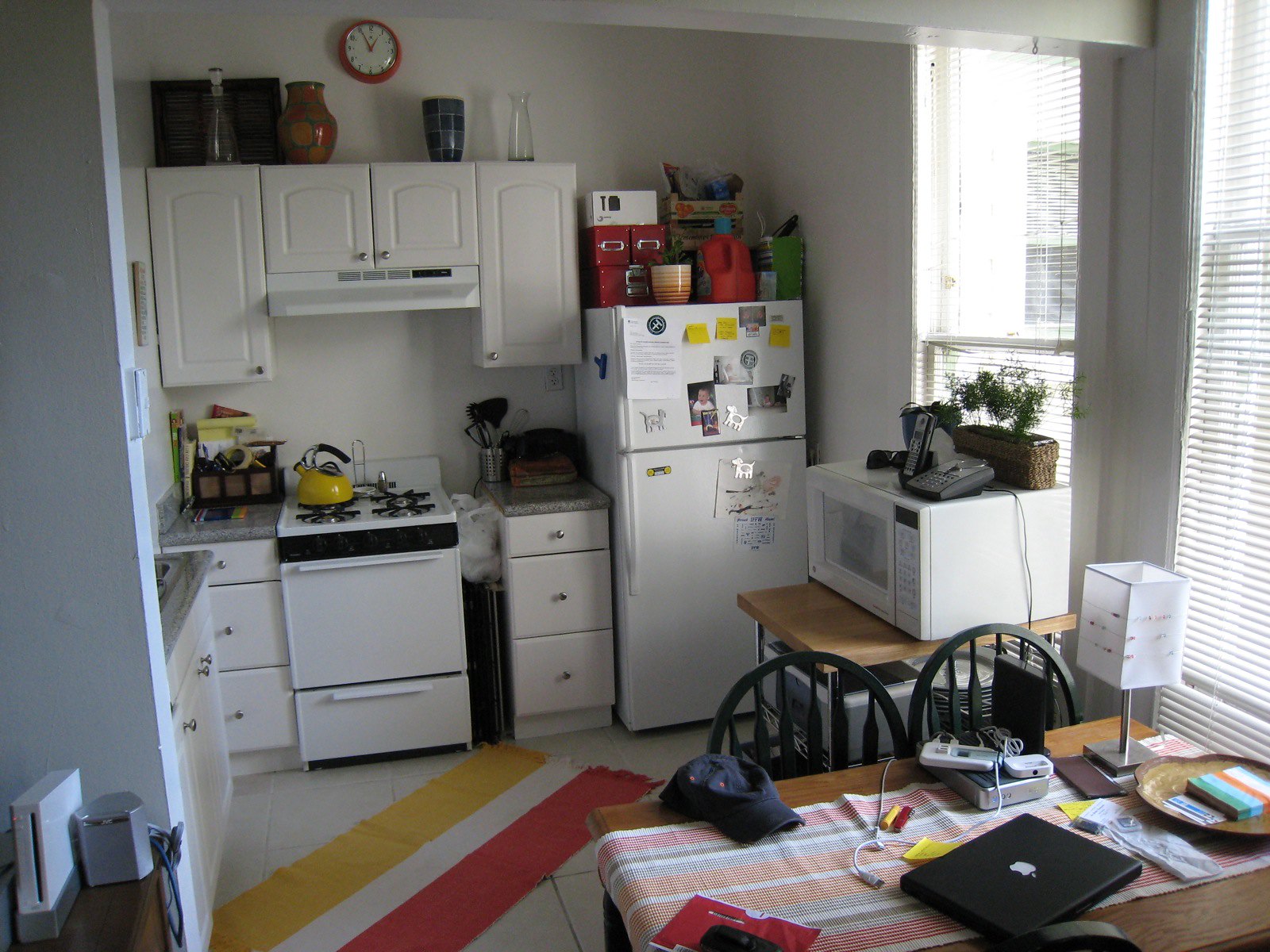This image captures a cozy, L-shaped small apartment kitchen. The refrigerator is positioned against the wall adjacent to sleek white cabinets, which provide a clean and modern look. On top of the cabinets, various decorative vases add a touch of personality to the space. Above the cabinets, a vibrant red clock adds a pop of color and an element of fun. Centered between two windows, a table holds a large microwave, highlighting the practical use of space. The table also serves as a multifunctional surface, displaying a MacBook, a lamp, several hats, and an assortment of post-it notes, indicating a blend of work and daily life activities in this charming kitchen.